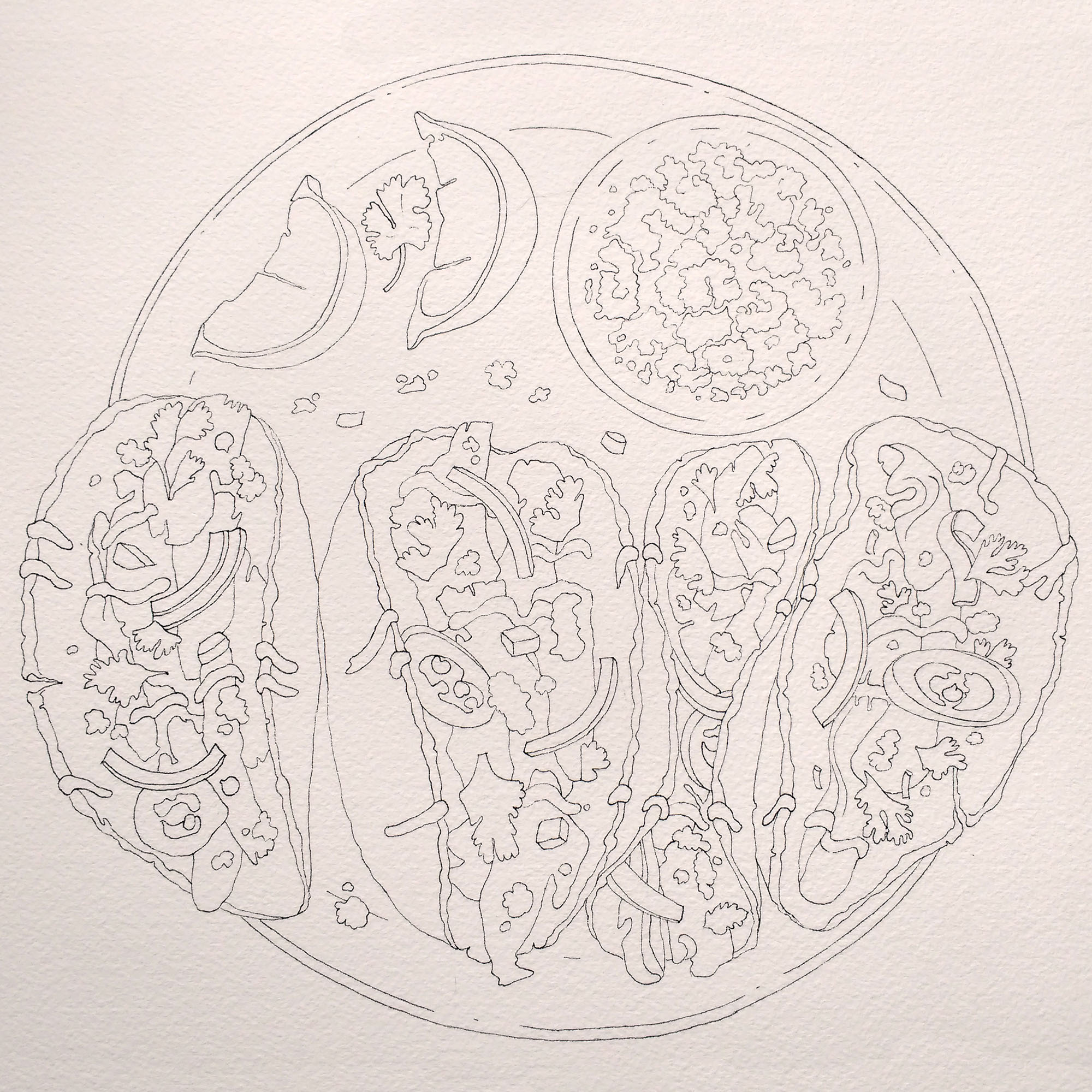The image is a detailed pencil sketch on what appears to be textured, beige or pinkish cardboard or drawing paper. The sketch prominently features a circular arrangement containing various food items. Within this circle, there are multiple tacos, specifically three or four, illustrated in various states of being filled or eaten. The tacos are depicted with ingredients such as lettuce, meat, onions, and possibly slices of green onion, with one taco noticeably cracked and another partially consumed. Additionally, the upper right side of the circle showcases a round plate laden with small, irregularly shaped pieces, while to the left, a couple of watermelon slices flank a parsley leaf. The entire composition, rendered in faint, nuanced pencil strokes, lacks any artist's signature or date.